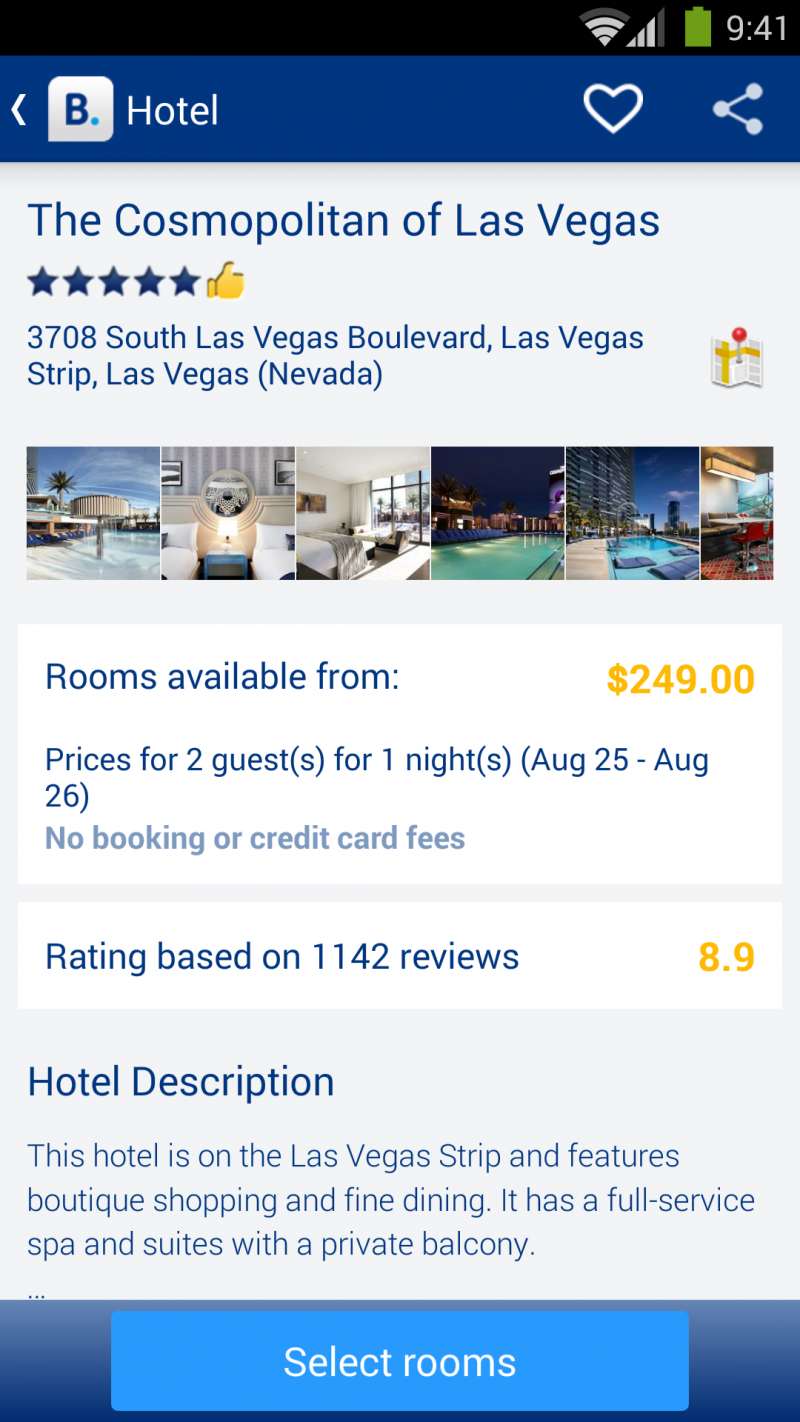**Screenshot of Hotel Booking Page**

The screenshot depicts an interface from a hotel booking website, shown on a booking screen. At the very top of the screen, there is a white box featuring the letter "B" with the word "hotel" in white lettering beside it. The body of the app page has a light blue background.

Prominently displayed at the top of the page is the hotel name, "The Cosmopolitan of Las Vegas", accompanied by five gold stars and a thumbs-up emoji, indicating positive reviews. Directly beneath the hotel name, the address is displayed with a small map icon featuring a pin drop to its right, suggesting a clickable map feature for location details.

A horizontal row of square thumbnail images showcases various views and amenities of the hotel, with an option to scroll through additional pictures.

Further down, under the section titled "Rooms available from", the starting price of $249 is highlighted in large yellow font. Accompanying this, a line states that the price is for two guests for one night, specifically from August 25th to August 26th, emphasizing that no booking or credit card fees are required.

The rating of the hotel, based on 1,142 reviews, is displayed at the bottom of the main content, showing an impressive score of 8.9 in yellow. Below this, a section titled "Hotel Description" appears but remains truncated in the screenshot.

At the very bottom of the page, a blue footer contains a prominent light blue button labeled "Select Rooms", inviting users to proceed with the booking process.